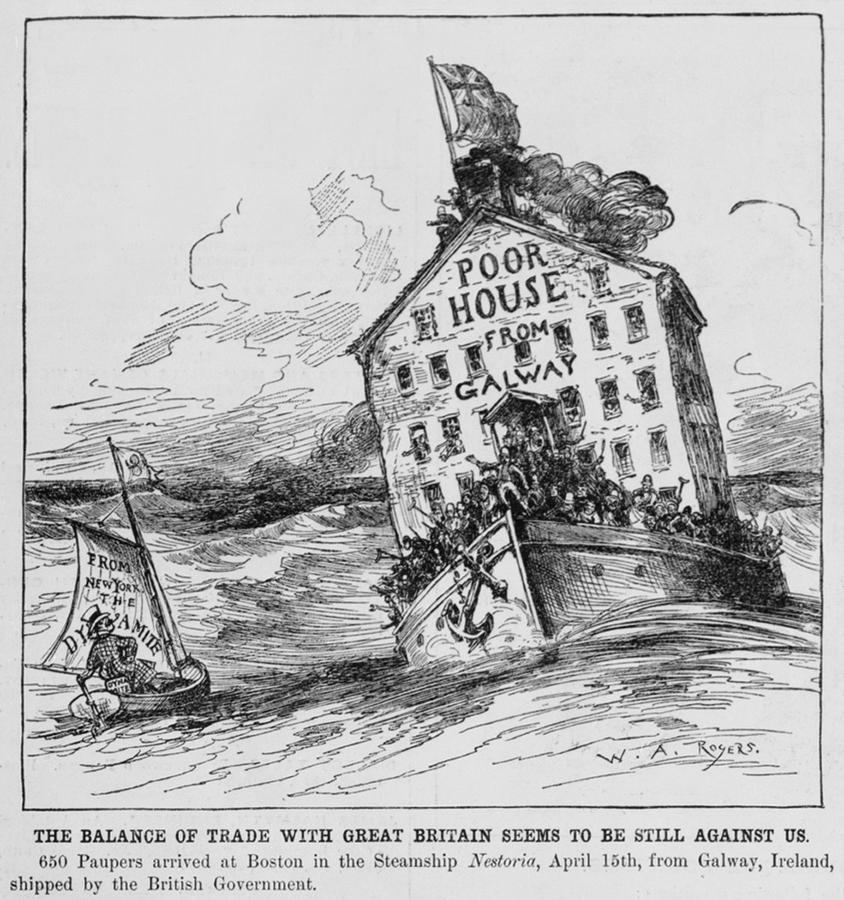The image is a black-and-white illustration from an old newspaper or magazine, depicting a stormy sea with a large, distressed boat that appears to be capsizing. This boat features a four-storey building labeled "Poor House from Galway," complete with a Union Jack on its chimney, belching smoke. The boat is overcrowded, with masses of people packed at the bow, and navigates murky, rough waters. In front of the main boat, there's a smaller lifeboat containing a solitary wealthy figure in a top hat and checkered suit, possibly steering and smoking a pipe. The obscured text on the sail of this smaller boat reads, "from New York," and partially "the dynamite." The artist's signature, W.A. Rogers, is visible at the bottom right of the image. Beneath the illustration, a text passage reads: "The balance of trade with Great Britain seems to be still against us. 650 paupers arrived at Boston in the steamship Nestoria, April 15th from Galway, Ireland, shipped by the British government."